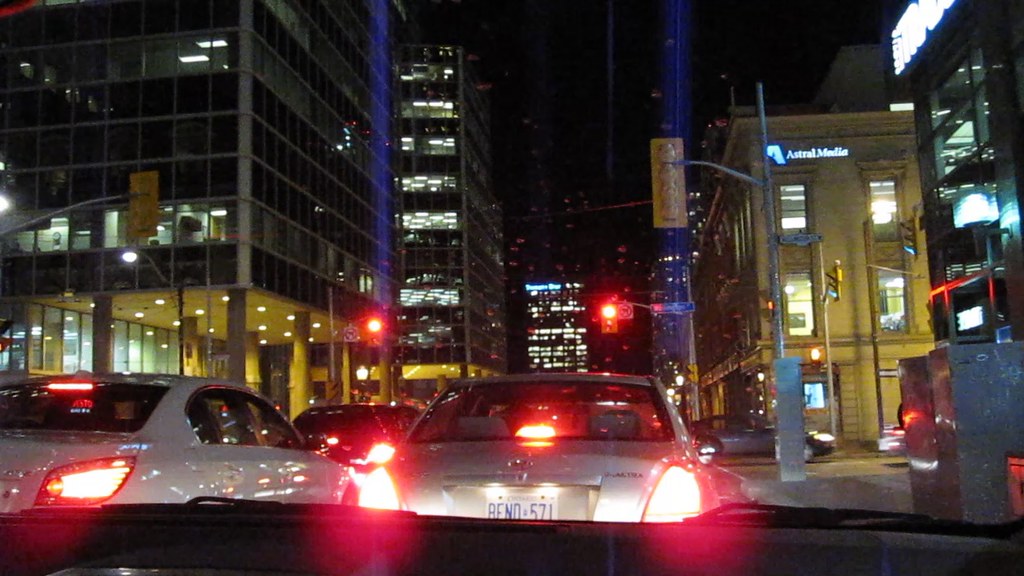The view from the passenger side of a car through the windscreen captures a busy junction in an American city. On the left, towering glass skyscrapers reflect sunlight, while on the right, a stone brick building bears the sign for Astral Media. All traffic is halted at a red traffic light, with several sedan-type cars in shades of white and beige lined up ahead. The scene is illuminated by a multitude of light reflections from the skyscrapers and car lights, with rear headlights and brake lights prominently glowing red, adding a vibrant touch to the urban landscape.